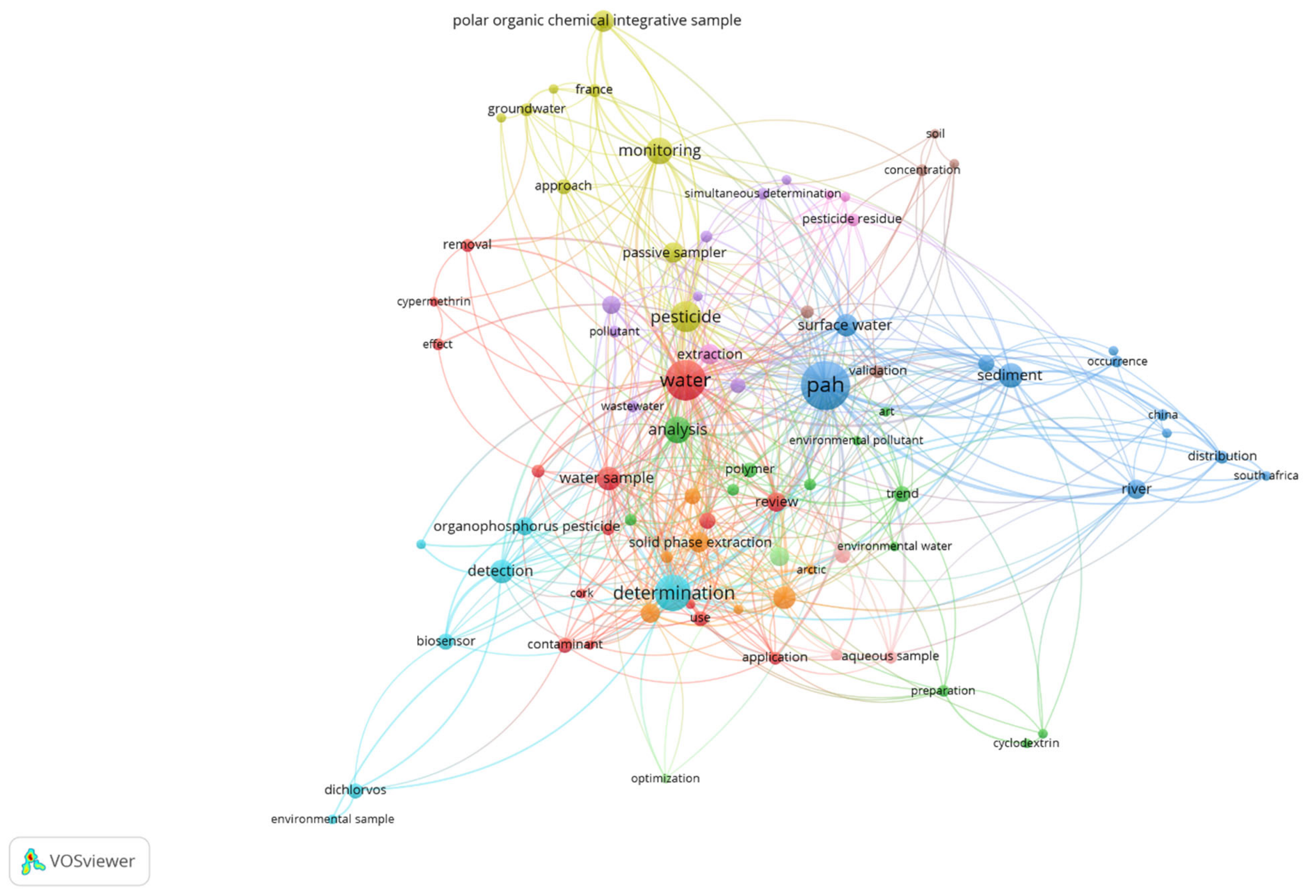The image features an intricate web of interconnected words, each within color-coded circles. Dominating the center left is a large red circle labeled "water," while a prominent blue circle on the center right is marked "PAH." Surrounding these central nodes are numerous smaller circles in various colors, each linked by lines of the same hue. Near "water," associated terms include "wastewater analysis," "extraction," "pesticide," "pollutant," "passes," and "sampler." Around "PAH," you find words such as "surface water validation," "environmental pollutant," "trend," "sediment," "occurrence," "China," "distribution," "South Africa," and "river."

The color distribution includes yellow circles at the top (e.g., "polar organic chemical integrative sample"), blue circles to the right (e.g., "distribution," "occurrence," "environmental samples"), green circles and their connections at the bottom right (e.g., "preparation"), orange circles under "water," and turquoise circles at the bottom left. A distinct rectangular box at the very bottom left contains the term "VOS viewer." The layout resembles a tangled spiderweb, visually representing the complex interconnections among these environmental topics.